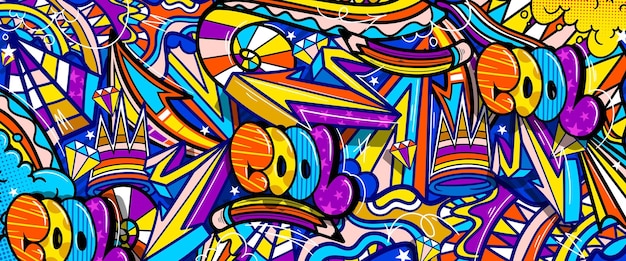This vibrant piece of graffiti art is bursting with an array of bright colors including purple, orange, blue, yellow, red, and pink. The word "cool" appears three times, each time with the letters C, O, O, and L individually colored in orange, yellow, blue, and purple respectively, adorned with pink stars on the L. The image is filled with various eclectic elements such as crowns, designed in rainbow hues including purple, red, yellow, and blue, as well as bent pencils that transition through purple, orange, and yellow with blue near the eraser. There are intricate details like sunglasses, diamonds blending yellow, purple, orange, and white, and a multitude of shapes including triangles, zigzagging lines, and patterns like polka dots and stripes. This intricately detailed and bustling artwork invites viewers to closely explore and discover the many repeating and unique elements woven throughout.